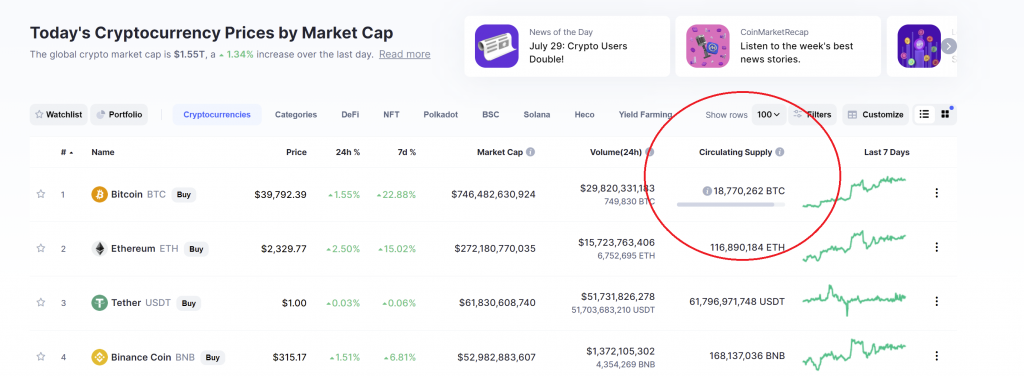This is a screenshot of a cryptocurrency tracking website or application. At the top left of the screen, black text reads: "Today's Cryptocurrency Prices by Market Cap." Below this, in gray text, it states: "Global Crypto Market is 1.55 Trillion, a +1.34% increase over the last day," with "+1.34%" highlighted in green. The main section displays a list of different cryptocurrencies along with their current prices. 

- **Bitcoin** is priced at $39,792.39.
- **Ethereum** is priced at $2,329.77.
- **Tether** is priced at $1.00.
- **Binance Coin** is priced at $315.17.

Adjacent to these prices are percentage changes indicating the fluctuations over the last 24 hours, showing all cryptocurrencies have increased in value. Further to the right, the changes over the past seven days are also shown, with each cryptocurrency exhibiting positive growth.

Additional statistics are provided, including the market cap, 24-hour trading volume, and circulating supply for the last seven days. The circulating supply statistic is emphasized with a red circle.